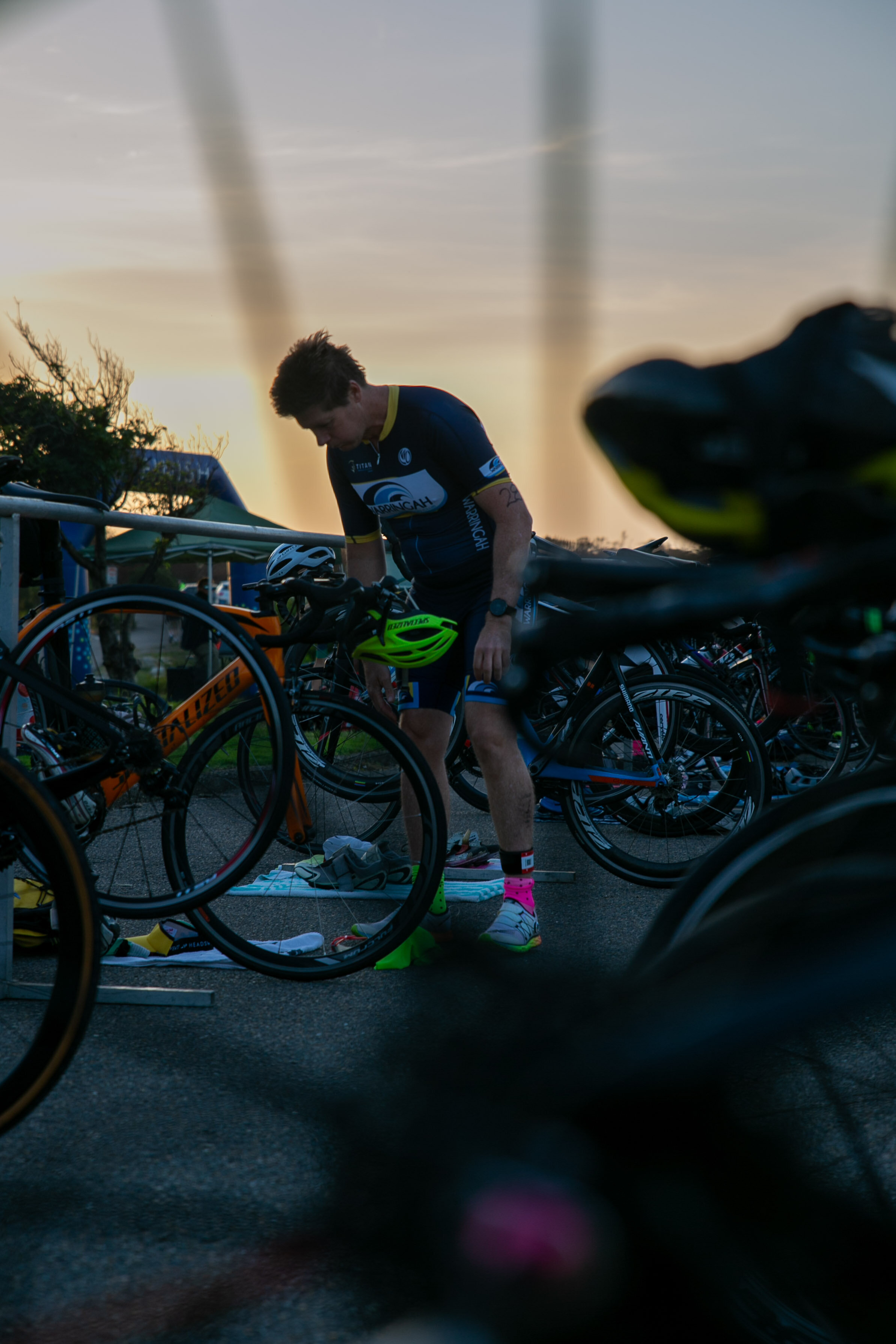In this portrait-oriented image, the focal point is a man dressed in typical biker gear, standing next to his bicycle. His outfit includes tight black biker shorts and a matching spandex shirt with yellow accents around the neck and arms, and a white bar featuring blue imagery and text on the front. Strikingly, he wears mismatched socks—one pink and one neon yellow—and white tennis shoes. In his hand, he holds a neon green helmet. The man is leaning slightly, intently inspecting his bike, which features notable orange details and some black writing. The background is filled with rows of bicycles stacked in bike racks, indicating a busy, communal bike area. The photographer has creatively taken the picture through the spokes of a bicycle wheel, adding an interesting visual element that partially obscures the lower right part of the image. Scattered around this area are various clothes and shoes. The setting features a mix of natural elements, with a few trees visible and a sky that transitions from blue to orange, suggesting either sunrise or sunset, casting a diffuse light on the scene.